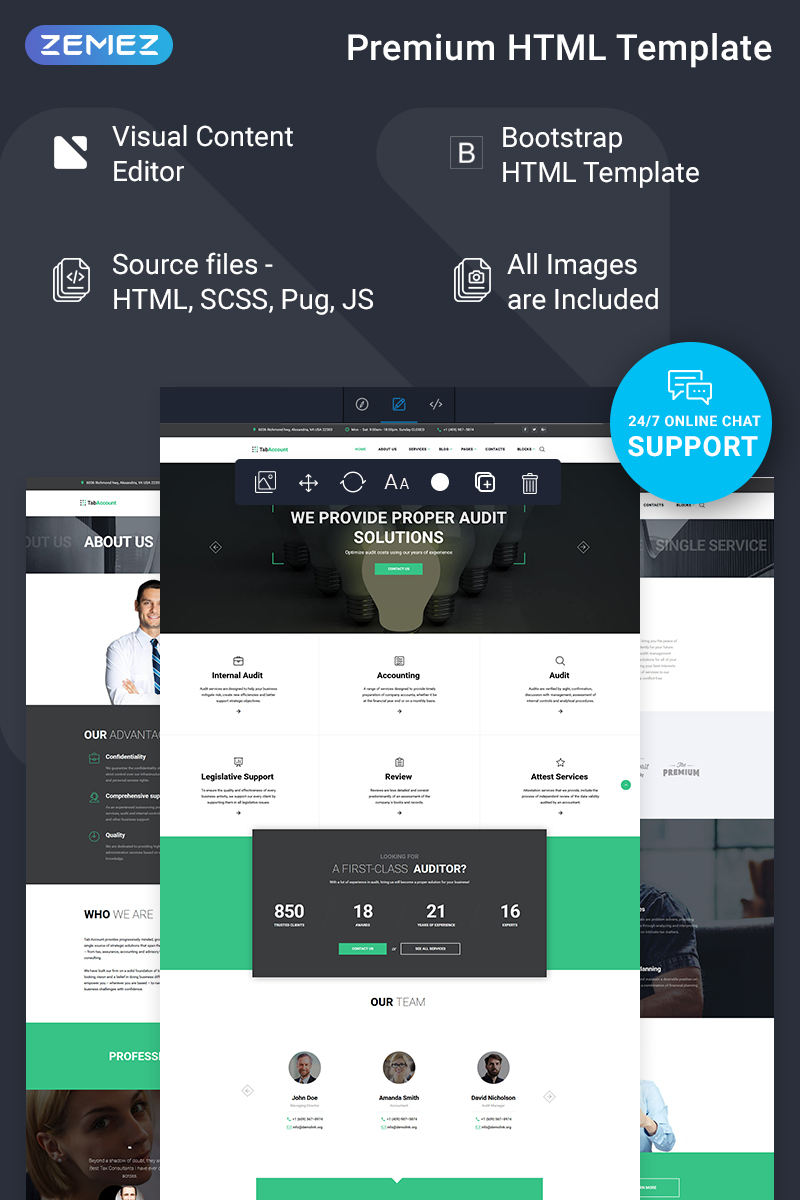**Detailed Caption for the Zemez App Screenshot:**

In this detailed screenshot of the Zemez app, we are introduced to Zemez, a premium HTML template platform. The screenshot highlights some of the key features and offerings provided by Zemez. It prominently mentions various aspects of the premium template, such as a visual content editor, and support for Bootstrap HTML. The source files available with Zemez include HTML, SCSS, Pug, and JS, ensuring a comprehensive and flexible development environment for users. All necessary images are included within the templates, significantly streamlining the design process by eliminating the need to search for visual assets.

The screenshot showcases a specific example of the template in use, displaying what appears to be the account tab, likely offering a representation of how different sections of a website can look using these templates. Zemez is not limited to a single template but provides a variety of options to cater to diverse design needs. An additional noteworthy feature highlighted is the 24/7 online chat support, making it convenient for users to seek assistance at any time. This service, along with the comprehensive inclusion of source files and images, positions Zemez as an ideal solution for users looking to start website development efficiently from scratch.

Overall, Zemez appears to be a robust and user-friendly platform aimed at simplifying the web development process with premium resources readily available and continuous support.